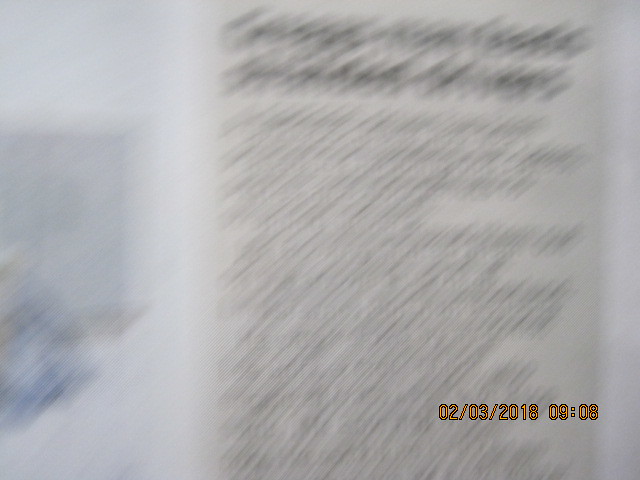This is a very blurry photograph of a white poster with illegible black cursive writing, possibly on a wall. To the left of the poster, there seem to be patches of light blue and darker blue colors, though their details are indistinguishable due to the blur. The foreground features a clear date and time stamp in the bottom right corner, displaying "02-03-2018" and "09:08" in yellow numbers with a black border around them. It is unclear whether the time is A.M. or P.M.